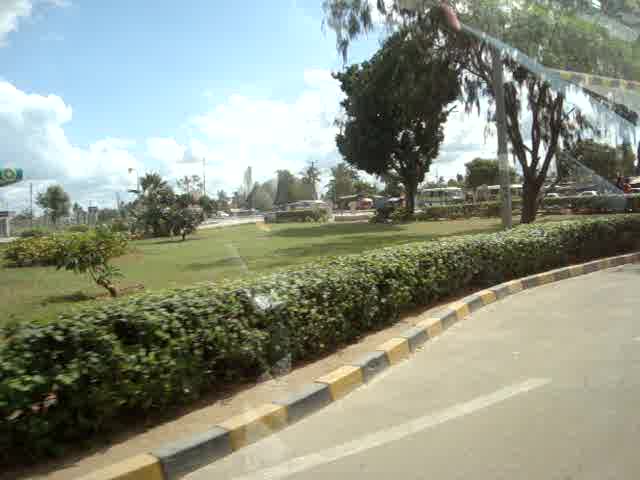This color photograph, taken from within a vehicle, captures a road that is about 10 to 20% wider than it is tall. The road features a noticeable S-like curve that begins from the lower left corner and meanders diagonally to about the middle of the right side of the image. The curve itself is bordered by alternating gray and yellow rectangular blocks, delineating a clear division between the roadway and the adjacent space.

To the left of this colorful curb, there is a row of dense green shrubs, followed by a well-maintained grassy area interspersed with leafy trees, akin to a park or golf course. The background reveals more trees and possibly small buildings. The sky overhead is a vibrant blue, speckled with white, puffy clouds, indicating a partly cloudy day with plenty of sunlight.

In the lower right-hand corner of the image, part of a concrete surface is visible, suggesting that the photo may have been taken in a parking lot. There is a distinct reflection visible in the upper right corner, further implying that the photograph was taken from behind a window, likely from inside a car. The perspective is akin to what one might see while looking out through a car windshield or side window, emphasizing the outdoor, daytime setting.